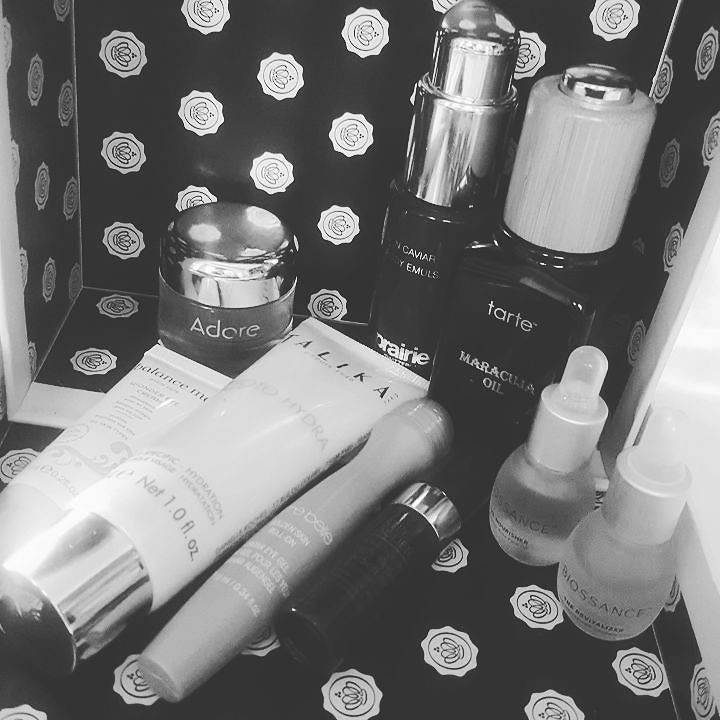This black-and-white photo showcases a collection of feminine products, primarily makeup items. The composition features a background with a gray border that extends down approximately a third to half of the image, framing the products within a black box. The box displays silver emblems, which are embossed and include a sideways crown with the top point facing right.

Inside the box, there is a visible lid on the left side, slightly open, allowing light to enter from the left. Positioned at the top is a small glass jar with a silver lid, labeled "Adore" in silver lettering. To the right of this jar, there is a taller, slender spray bottle. The top half of this bottle is silver, tapering inward at the top, while the bottom half is black with some barely legible lettering at the top and "Prairie" at the bottom.

To the right of the spray bottle is a black bottle with a white cap and a silver tip. The front is labeled "Tarte Maracuja Oil" in silver lettering. 

In the foreground to the left, a white tube with black lettering lies diagonally from the bottom left to the top right. Adjacent to it, another wider white tube with a silver tip extends in a similar direction, with black lettering on its body.

Further to the right is a long, slender plastic stick, positioned diagonally left to right, with a clear roller ball tip and white lettering on the body. Next to it is a small black bottle with a silver cap, angled top right to bottom left. Completing the assembly are two small clear bottles with white caps, situated on the right side of the box, one placed slightly behind and to the left of the other. 

The meticulous arrangement of these makeup products within a structured, bordered frame gives the image a sense of organized elegance and minimalist aesthetics.